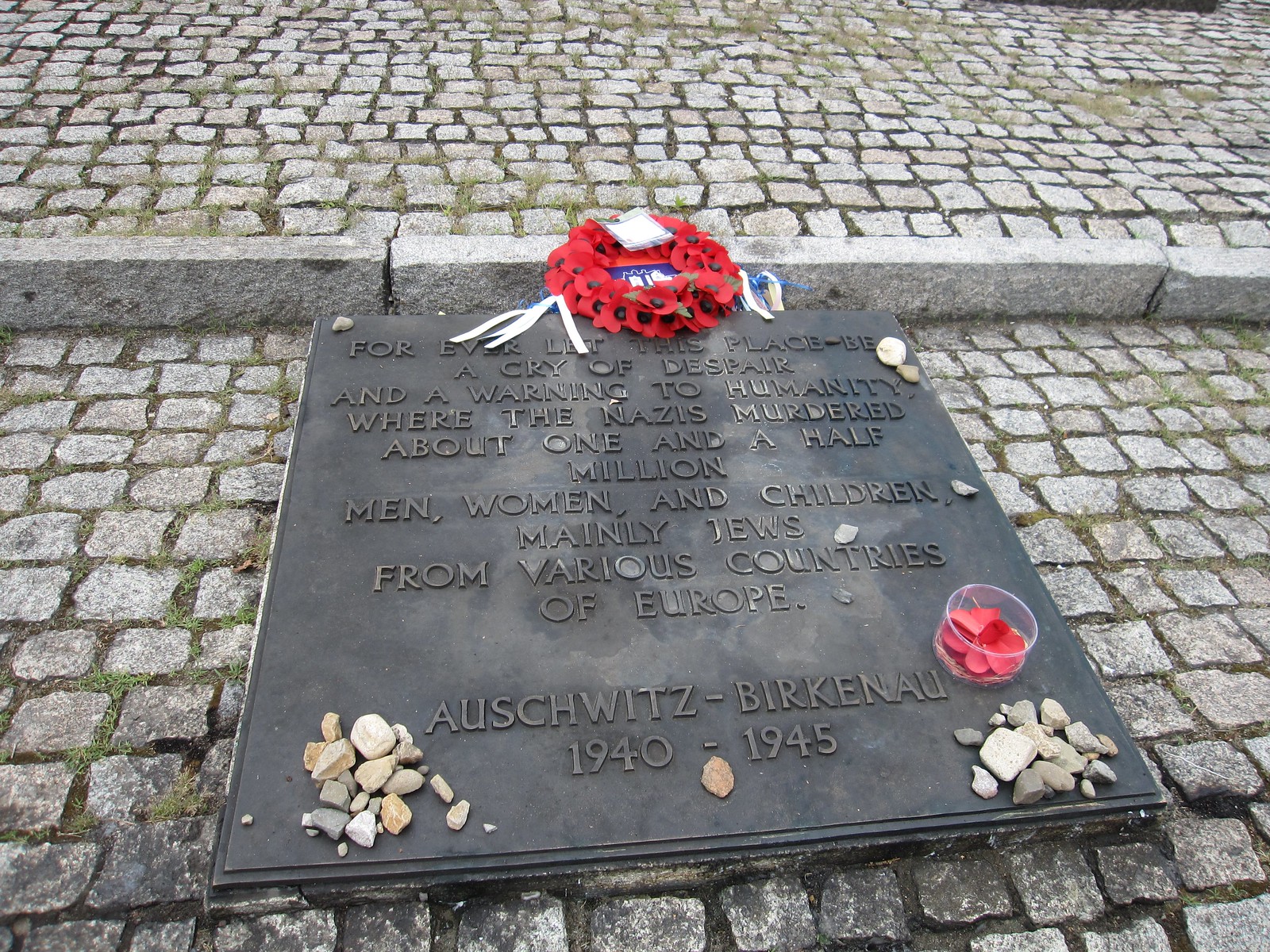The image depicts a detailed view of a flat tombstone or memorial plaque set on a very old stone pavement, with grey bricks weathered and adorned with tufts of grass growing between them. The plaque, made of metal or bronze, bears an inscription that reads, "Forever let this place be a cry of despair and a warning to humanity where the Nazis murdered about one and a half million men, women, and children, mainly Jews from various countries of Europe. Auschwitz-Birkenau 1940 to 1945." At the top, there is a floral arrangement featuring red flowers or poppies, accompanied by a red ribbon. Scattered around the bottom left and right corners are various stones and rocks. Additionally, a small plastic container with rose petals and a dried leaf are placed on the plaque. The perspective of the image suggests that it may be shot at an angle, giving an impression that the plaque is either lying flat on the ground or affixed to a wall.